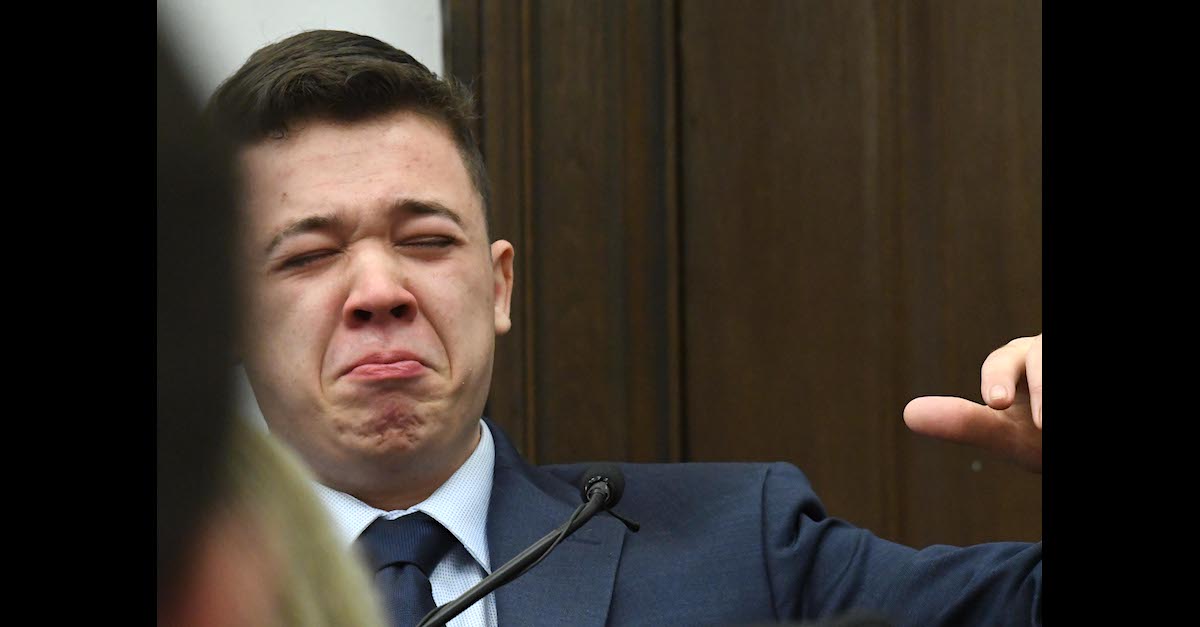This is a detailed image of Kyle Rittenhouse, a young Caucasian man likely in his late teens or early twenties, captured during a court session. He has short brown hair parted to the right side of his face. Dressed in a black suit with a crisp white collared shirt and a black tie, he is seated in front of a small black microphone. His left hand is visible, raised, and he appears to be making a contorted facial expression—his eyes are squeezed shut, and his whole face is scrunched up, indicating he might be about to cry. The background features a wooden panel wall with molding, and in the bottom left corner, there is a partial view of a blonde-headed individual. The overall setting suggests a formal or judicial environment, accentuated by the somber attire that resembles funeral clothing.